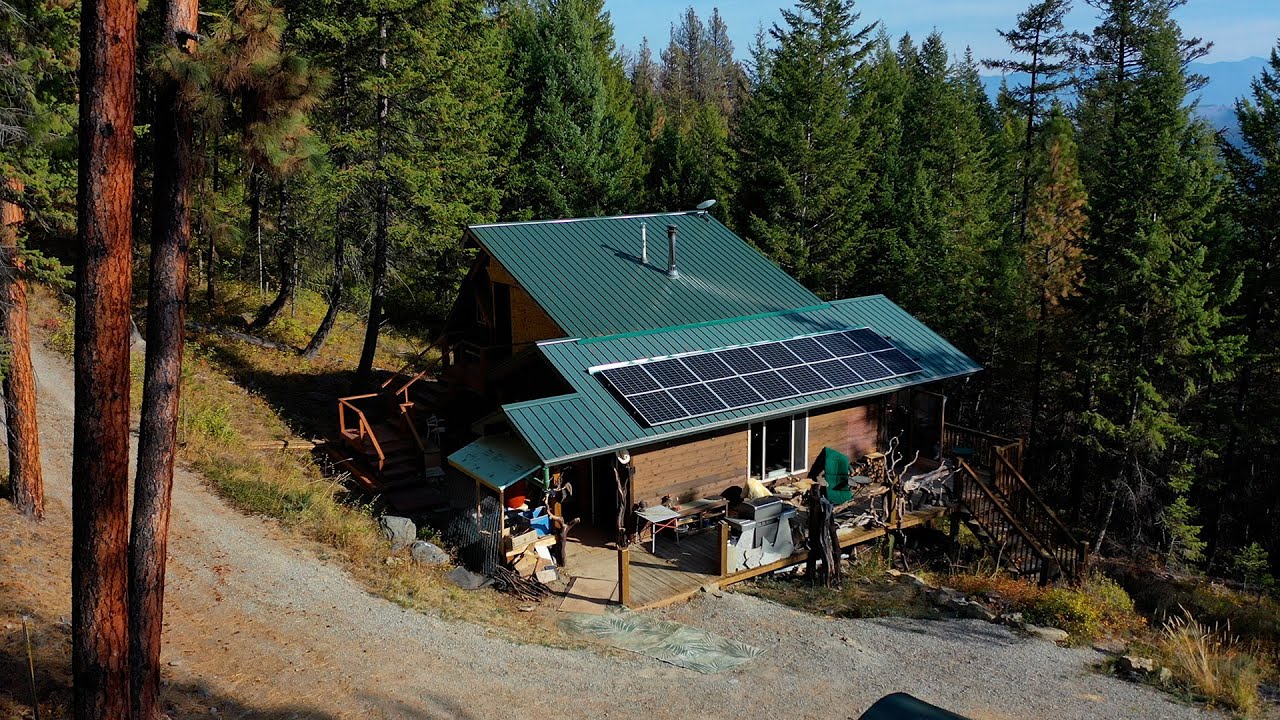The image depicts a rustic wooden cabin nestled in a dense forest of tall, dark green evergreen trees, captured on a bright sunny day. The overhead shot reveals the cabin's slanted dark green metal roof, adorned with a row of solar panels at the lower end. Two metal chimneys protrude from the top of the roof. A broad porch wraps around the cabin, cluttered with various furniture items and other belongings, adding to the lived-in feel. A long gravel driveway curves around the cabin, hinting at the possibility of a road nearby, although it doesn't seem wide enough for a car. The backdrop features a beautiful blue sky with sporadic clouds, further emphasizing the serene and secluded atmosphere.